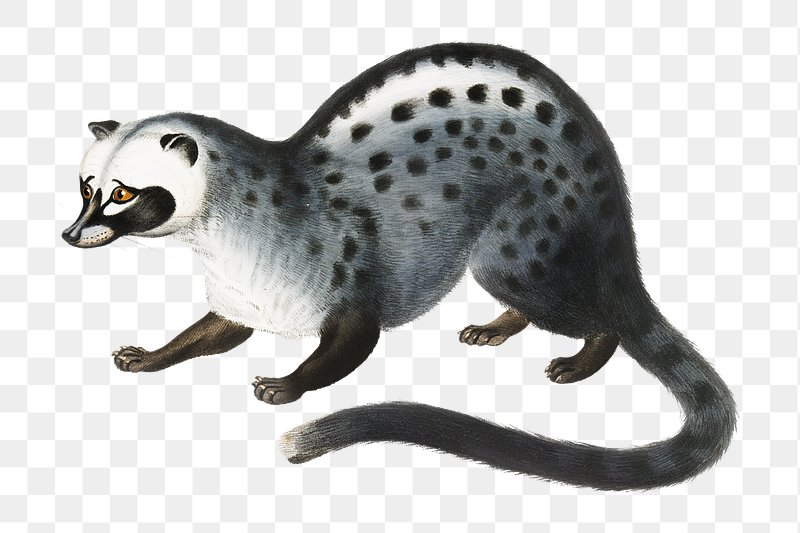The image is an illustration of an animal that appears to be a hybrid of a possum, raccoon, and perhaps a cat. The background features a white and light gray checkered pattern. The animal, which is on all fours and facing toward the left, has a white fur coat adorned with black spots and a dark gray body, accented with patches of white on its chest and back. Its head is detailed with a white face, tiny black ears, a thin brown and black snout, and expressive brown eyes that look to its right. The animal's legs are dark brown, equipped with claws, and it has a long, striped gray and black tail that curves toward the left of the image. The creature exhibits a somewhat concerned expression, possibly due to the intricate patterning of its fur.